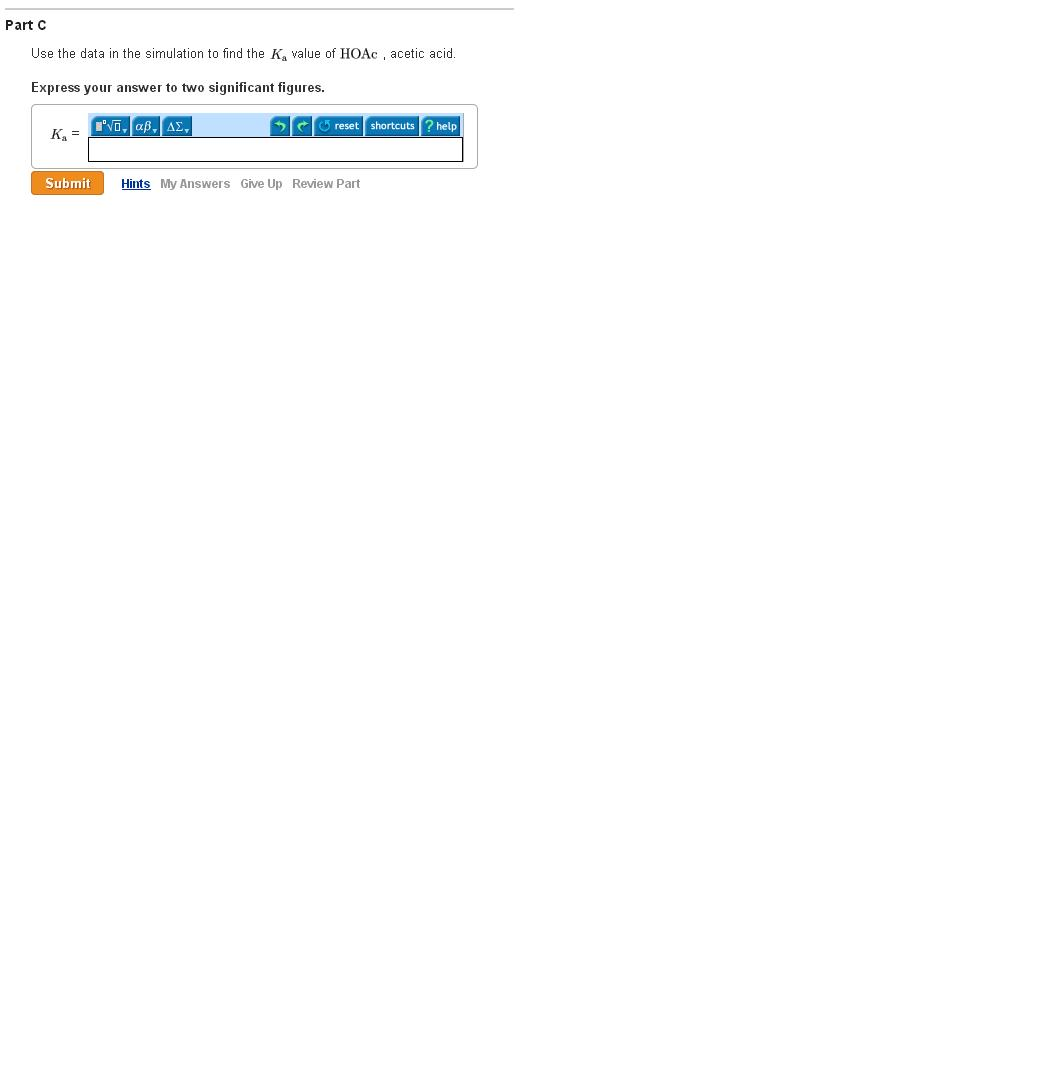The image is a detailed screenshot of a mathematical website interface, specifically focusing on a problem-solving section labeled "Part C." At the top, a very thin, light gray horizontal line stretches across the width of the image, separating the header from the content below. 

On a clean white background beneath this line, the top left corner features bold black text reading "Part C." Directly below it, in regular thin black font, is the instruction: "Use the data in the simulation to find the Ka value of HOAC, acetic acid." Below this, a smaller bold text further specifies, "Express your answer to two significant figures."

In the center of the image, there is a rectangular input area. On the left side of this rectangle, there is text reading "Ka equals," while the right side is populated with several blue buttons. These buttons feature various mathematical symbols and functions, including arrows representing undo, redo, reset, shortcuts, and help options. 

At the bottom of the input area, there is a prominent yellow "Submit" button with white text. To the right of this button, a blue hyperlinked text reads "Hints," followed by gray text stating "my answers." Continuing to the right, there is a "Give Up" button, and further right, a "Review Part" button.